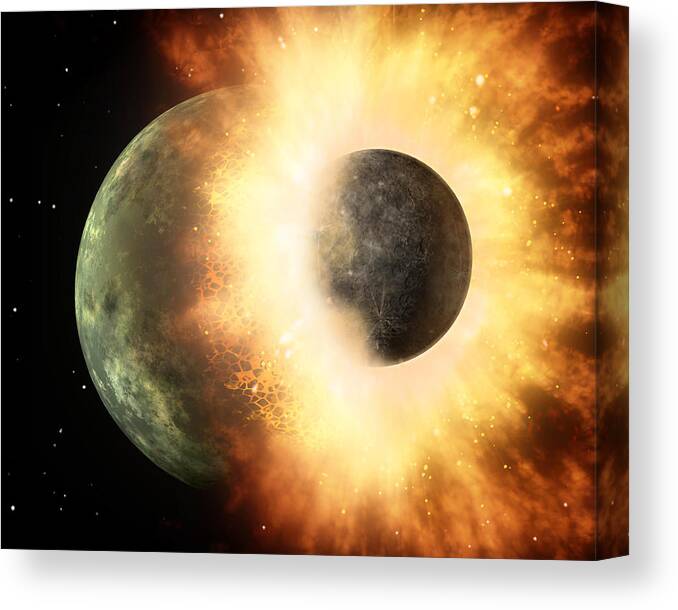This artwork, displayed on a slightly angled, three-dimensional canvas, captures a dramatic collision between two planetary bodies set against a black background speckled with tiny, white stars. The central focus is a larger, greenish-white planet with hues of light green, yellow, and dark green, being violently struck by a smaller, dark gray planetary body from the right. The impact causes an explosion of brilliant white, yellow, and red hues, creating molten cracks on the larger planet. This explosion forms a striking circular ring that spills off the edges of the canvas, adding to the dynamic nature of the scene. The overall image exudes a sense of cosmic chaos, with the planets and the explosion centered in the frame, vividly illustrating the cataclysmic event.